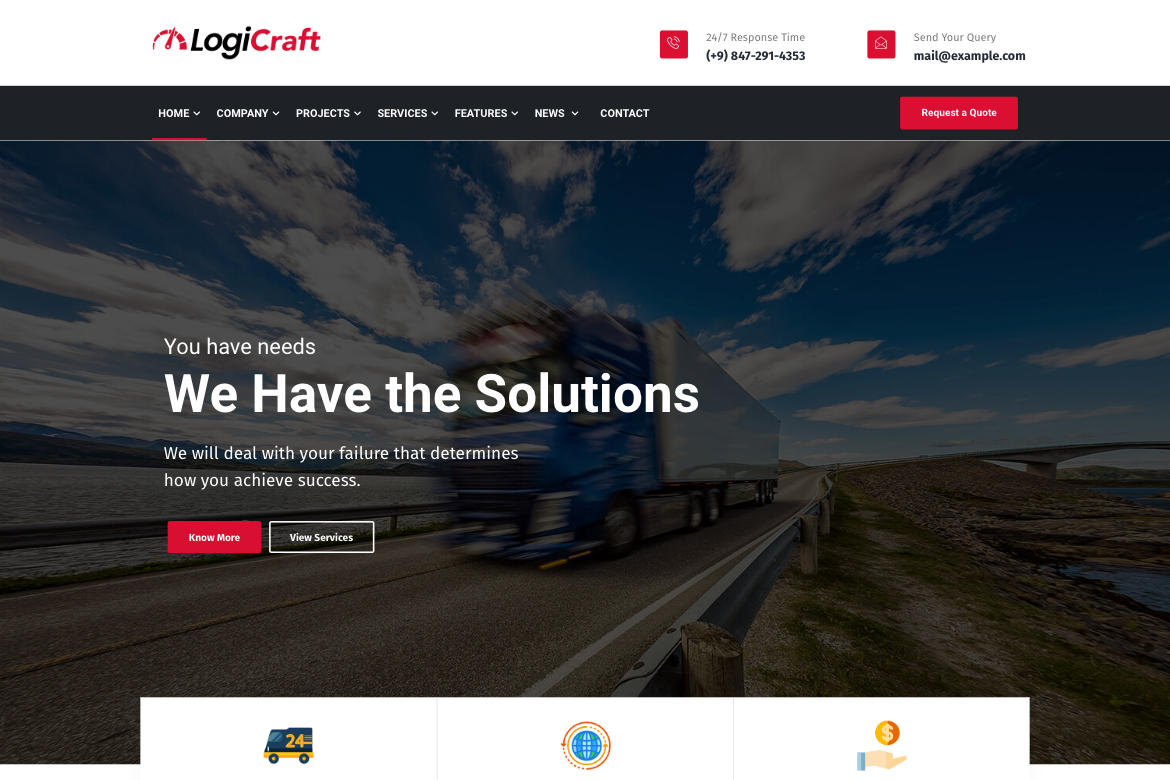The image features a visually distinctive top half with a white background and black text. Prominently displayed in the top section is the text "Logi" followed by "CRAFT," with "CRAFT" highlighted in red lettering. Below, in gray text, it states "24/7 response time," clarifying availability 24 hours a day, 7 days a week. A contact number, "(+9) 9847-293-4353," is listed in black, while the text "send me a query" appears in gray. An email address, "mail@example.com," is also featured in black.

A dark gray horizontal border separates this information from the navigation menu below. The menu is predominantly white with the word "home" underlined in red, followed by options such as "Company," "Project," "Services," "Features," "News," and "Contact." A notable red rectangle with white text invites viewers to "Request a Quote."

The lower half of the image depicts a truck in motion on a highway. The truck's cab is blue and white, and it appears to be speeding, resulting in a blurred effect. The highway is bordered by grass, dirt, and a small body of water to the right, with a bridge visible in the distance. The left side of the image also shows more bodies of water. White clouds dot the sky, completing the scenic backdrop.

Text overlays the image, stating in white font, "You have needs, we have solutions. We will deal with your failure, that determines how you achieve success." Below this motivational message is a red rectangle with the text "Learn more" in white. Additionally, there is a transparent rectangle with a white border, featuring the phrase "View Services" suggesting further action for more details.